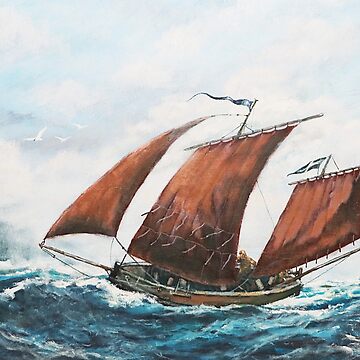The image depicts a detailed painting of a medium-sized wooden sailboat navigating through tumultuous seas. The boat, centered in the composition, is adorned with three prominent red sails and has a blue triangular flag at the top. The vessel, estimated to be around 20 feet long, appears to be expertly crafted with a brown, rustic hue that complements its sturdy construction. In the background, the sky is painted in a soft, pale blue with dense white clouds, adding to the dramatic atmosphere of the brewing storm. The dark blue sea features violent, choppy waves capped with white foam, suggesting a challenging voyage. A solitary figure with a blonde ponytail is visible on the deck, steering the ship amidst the chaos. Surrounding the vessel are seagulls, with at least three clearly depicted soaring in front of the sailboat, enhancing the maritime theme of the artwork. The overall scene is rich with dark tones and intricate details, showcasing the artist's dedication and skill in capturing the essence of seafaring adventure.